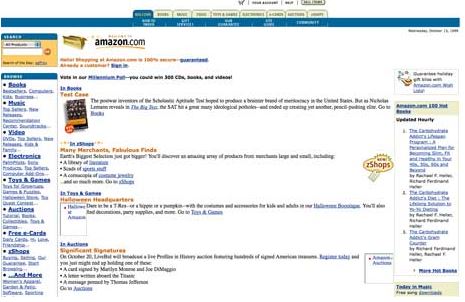The image depicts a page from Amazon.com with very low resolution, making most of the details difficult to discern. At the top, there are navigation tabs, but the text on these is unreadable due to the poor quality. The Amazon.com logo is prominent and clear, positioned near a small, fuzzy yellow or off-white band. Below this, there is a turquoise band with a blue tab, followed by more white sections containing additional items, although the specifics are too blurry to identify.

On the left side, a search bar is visible, and directly to its right, the Amazon logo is situated with the text "Amazon.com." Below the search bar, a list in blue bulleted points includes categories like books, music, videos, electronics, something related to games, auctions, an undiscernible term, and a 'more' option.

Beneath the Amazon logo, there is another piece of text that reads “test case,” and an indistinguishable graphic that vaguely resembles a device like a computer or calculator, though the resolution is too poor to confirm the precise details.